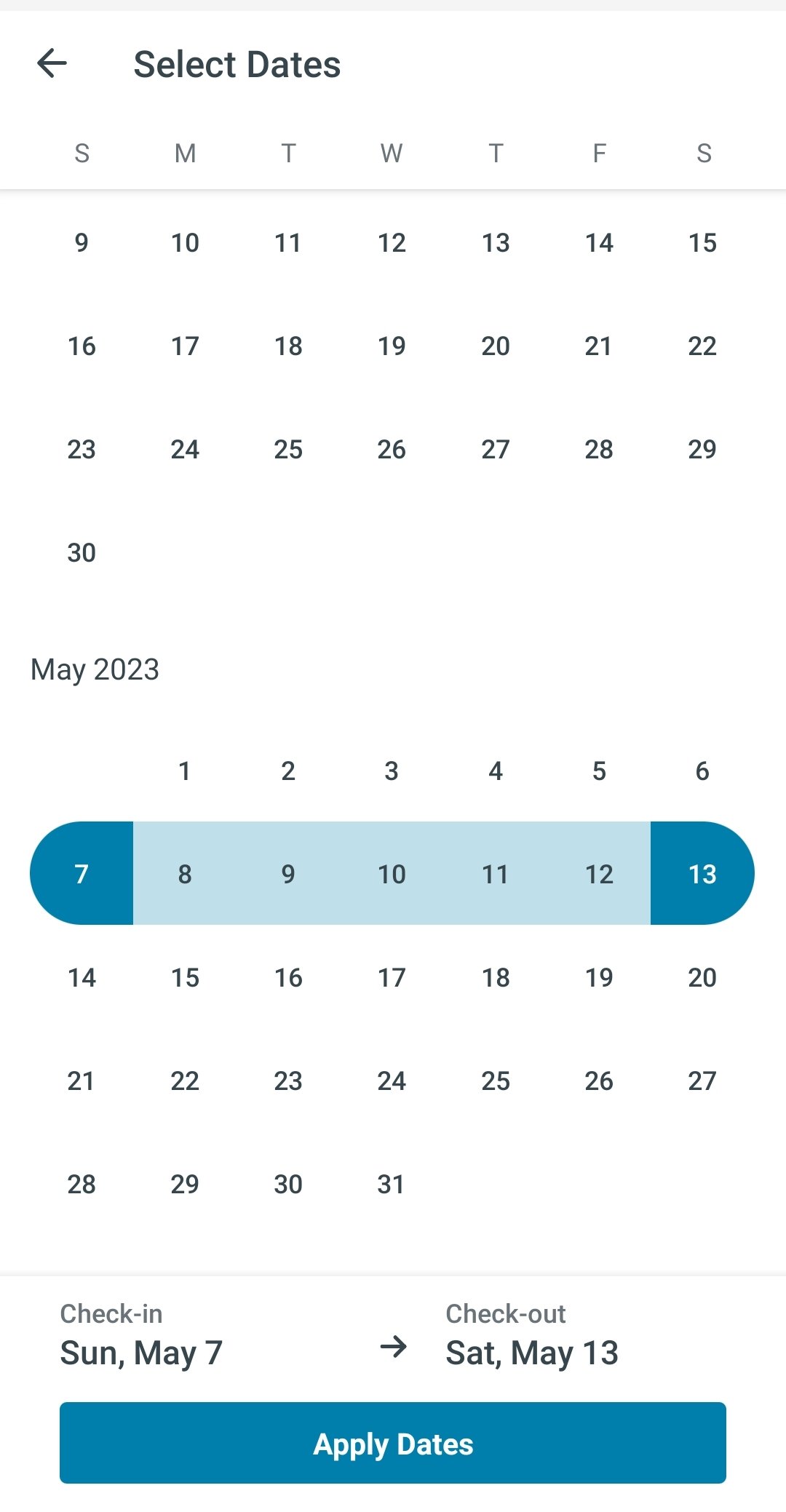The image displays a digital calendar interface for selecting reservation dates. At the top, there is a back arrow button. The calendar grid includes the days of the week: Sunday, Monday, Tuesday, Wednesday, Thursday, Friday, and Saturday. Specific dates are displayed, starting from the 9th to the 30th of April 2023, and from the 1st to the 31st of May 2023. The selected check-in date is Sunday, May 7th, and the check-out date is Saturday, May 13th. At the bottom, there is an "Apply Dates" button to confirm the selection.